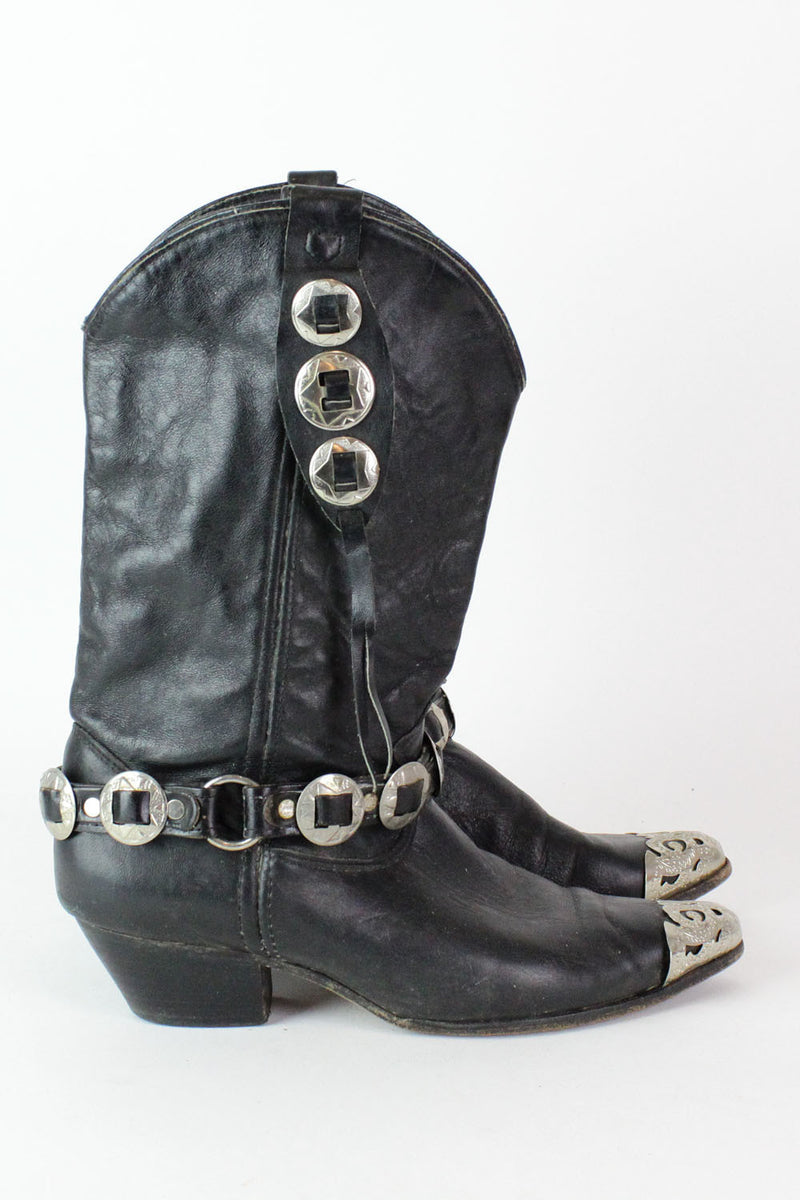The image is a rectangular-shaped photo oriented vertically, featuring a pair of black leather boots that stand out against an off-white background. The boots are positioned facing to the right and show clear signs of wear, with evident creases around the toes and wrinkling along the legs. They are crafted from aged leather, appearing slightly dirty and in need of cleaning or repair. Each boot features distinctive silver-plated toes, adding a shiny, sparkly touch to their rugged, cowboy-boot-like fashion design.

A notable detail is the presence of two black leather straps on each boot. The first strap starts at the ankle, circles around the front side, and is held in place by a silver steel ring at the back. It is adorned with several silver medallions and buckles, suggesting they can be tightened for a better fit. The second strap descends from the top of the boot to the ankle on the outside, embellished with more silver discs. Additionally, there is visible stitching on the other side of each boot. The boots also feature a small wedge heel, approximately one to two inches high, adding to their stylish yet functional appearance. They stand about one to two feet tall in total.